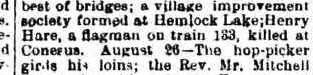This image shows a very pixelated, low-resolution scan of a text excerpt, likely from a book, newspaper clipping, or magazine article. The background is white, with black text arranged in five horizontal rows going down vertically. The font resembles an older typewriter style, possibly Times New Roman, featuring varying character widths indicative of an electronic typewriter. Although blurry, the text reads: "Best of Bridges; a village improvement society formed at Hemlock Lake; Henry Hare, a flagman on train 183, killed at Cornarus, August 26 - the Hoppicker Girls, his loins; the Reverend Mr. Mitchell." The left-hand side of the text is partially obscured, cut off from view. No other colors or defining markings are visible on the object.